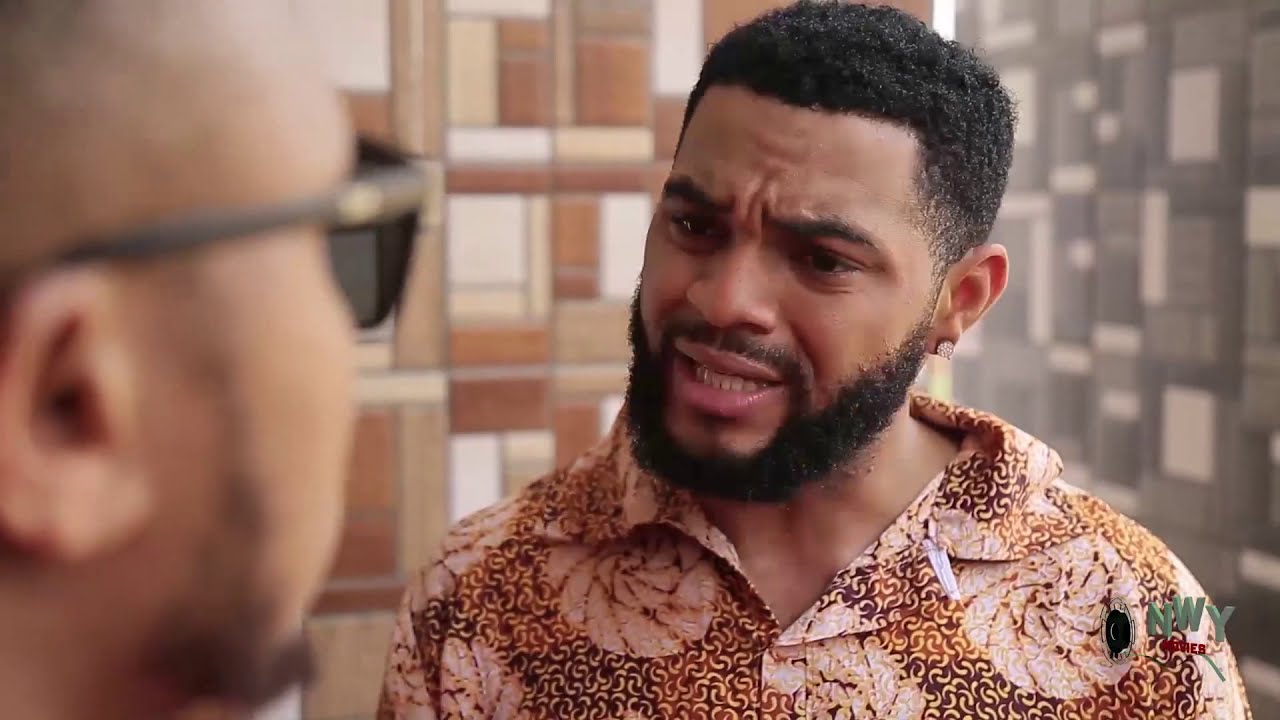In this detailed scene, we observe two men engaged in what appears to be an intense conversation. The focus is primarily on a light-skinned Black man in the background, who sports well-groomed black hair, a full beard, and a mustache styled into a Fu Manchu. His expression suggests he is upset or questioning something, with his mouth slightly open, revealing his bottom teeth. He wears a brown, orange, and pink floral-patterned button-up shirt that complements his studded earrings. 

The person he's speaking to is closer to the camera and slightly out of focus, showing only the right side of his face. This man also appears to be Black and is wearing sunglasses, with sideburns that transition into a lightly grown beard. Both men are framed against a geometric patterned wall comprising rectangles and boxes in shades of gray, white, brown, and beige.

In the bottom right-hand corner of the image, there is an overlaid text displaying the letters "NWY" and the word "series" beneath it, hinting that this could be a scene from a TV show or movie.